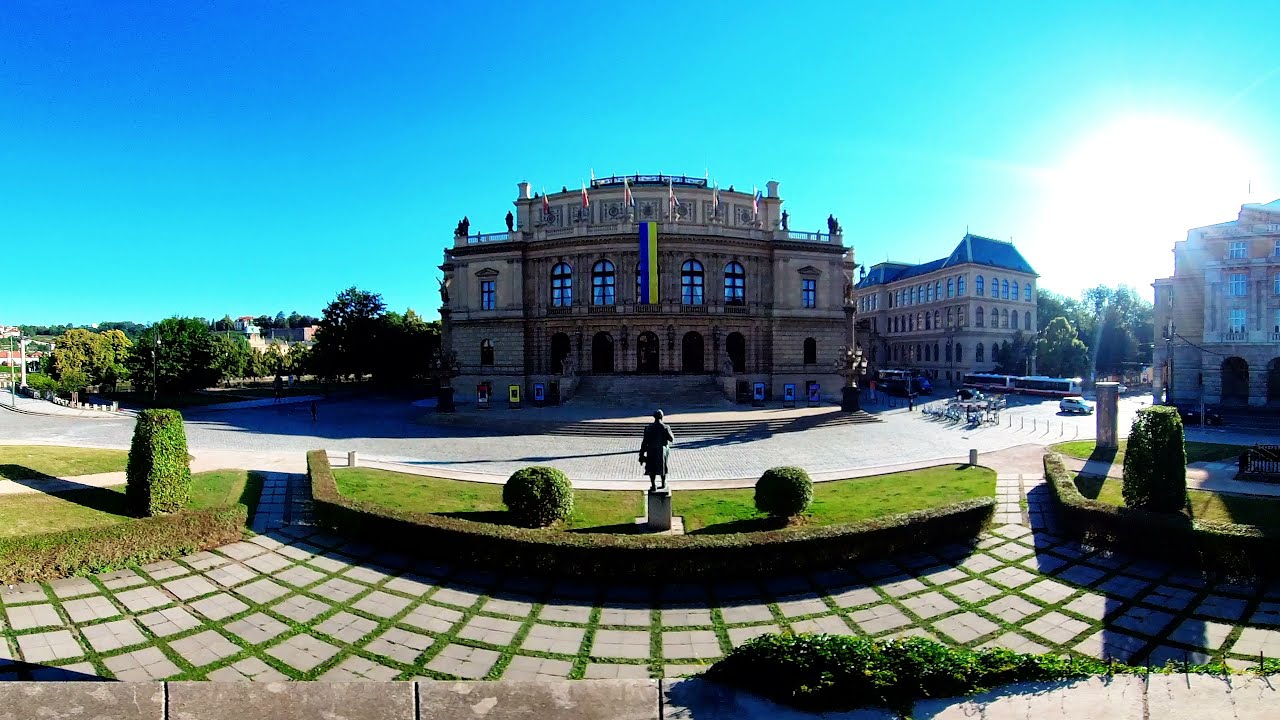The image is a stunning photograph of a historic, European-style building that resembles a castle or government building, possibly linked to a college or palace. The main structure is a grand three-story construction made of tan stone, featuring a sophisticated facade with five rounded, dome-shaped entryways. Draped centrally on the building is a prominent blue and yellow flag, which could be Ukrainian or Swedish. Surrounding the building, the gray cobblestone pavement transitions into a manicured courtyard adorned with meticulously shaped green shrubs and bright green grass. In front of the main building stands a statue of a man holding a book, wearing a long coat. To the right of the building are additional stoic, significant-looking structures, enhancing the historic feel. The photo captures a clear, bright day with a brilliant turquoise sky, a radiant white sun in the top right corner, and a mix of colors including green, blue, gray, black, white, yellow, brown, and tan. The composition is free of pedestrians, lending a serene and majestic atmosphere to the scene.